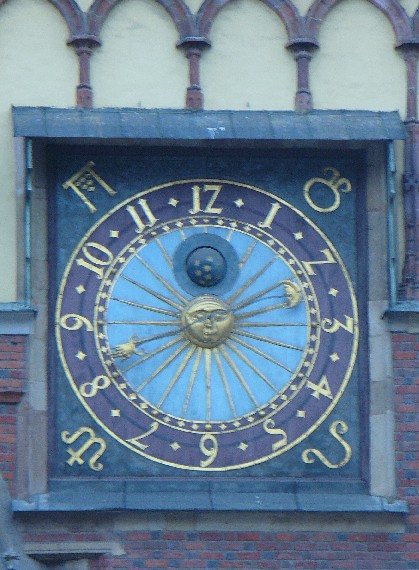This image showcases the side of an architecturally intriguing building, which embodies a Gothic-style aesthetic with medieval influences. The structure features a tan stucco façade complemented by elegant brass-like arches intricately woven into the building's design. The lower half of the building is accented with brickwork, adding to its historical charm.

The focal point of the image is a detailed and vibrant clock face set into the building. The clock, framed in a square, exhibits a mesmerizing blend of blue and purple hues. At its center is an ornate depiction of a celestial body, resembling either a sun or moon face. The clock's hands are golden, pointing gracefully at golden numbers set against the purplish background. Surrounding the clock are four golden symbols, positioned at the corners: one above the 1, between the 4 and 5, between the 7 and 8, and between the 10 and 11, each add a touch of mystique.

The architectural style of this building could be interpreted as influenced by Eastern European or Oriental designs, given its intricate details and exotic flair.